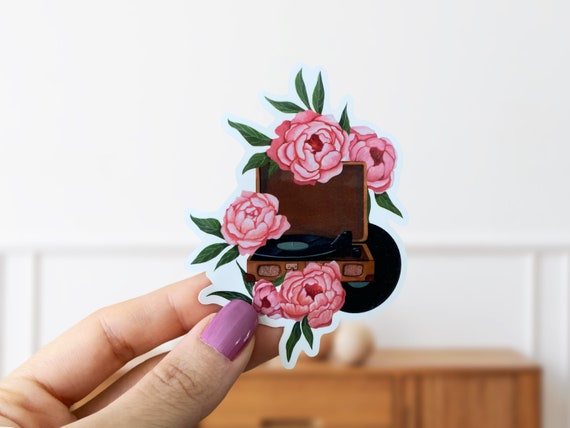A detailed photograph captures a white woman's left hand emerging from the lower left corner of the frame, holding a small, intricate object. Her nails are meticulously painted in a shiny, lavenderrish-purple color, highlighting her well-manicured fingers. The object she grasps appears to be a decorative magnet or trinket, prominently featuring an old-fashioned wooden phonograph or turntable with its lid open. A vinyl record and its arm are positioned as if playing music. Encircling this nostalgic centerpiece are five delicate pink roses, each adorned with two or three green leaves. The backdrop is out of focus but reveals a white wall and the faint outline of a brown wooden table, ensuring the hand and its held ornament remain the central focus of this composition.